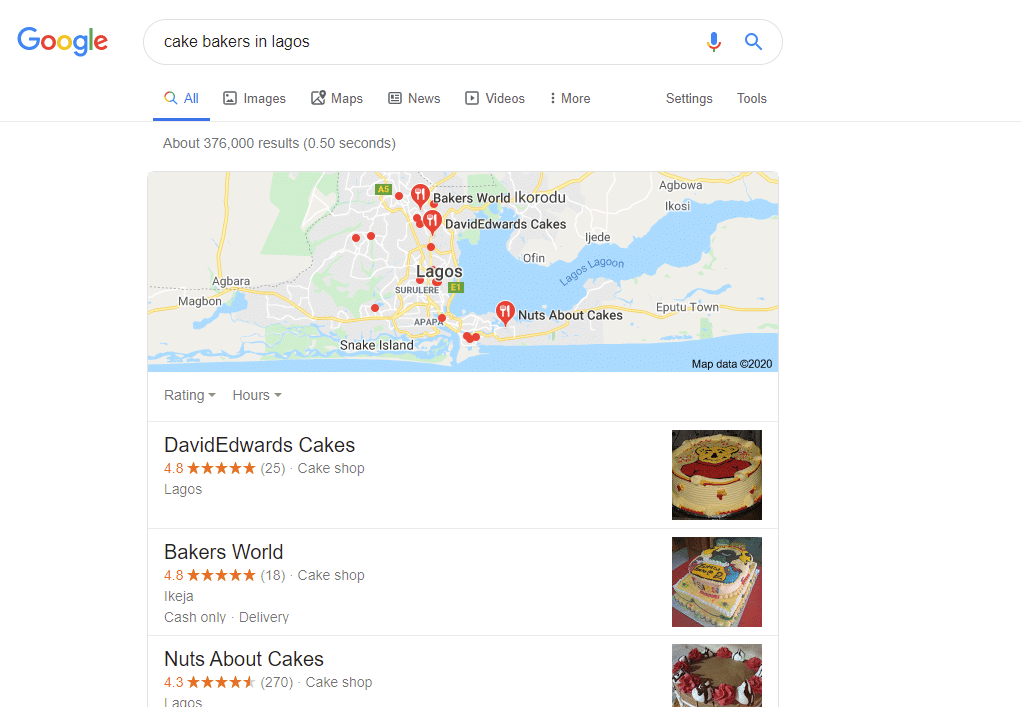A person is conducting a Google search on their device. The screen has a clean, all-white background. At the top left corner, the iconic, colorful Google logo is displayed, with letters in blue, red, yellow, and green. To the right of this logo, there's a search bar with the text "cake bakers in Lagos," typed in black. Adjacent to the search bar on the right, there are a blue search icon and a blue voice search icon.

Beneath the search bar, the standard Google navigation options are listed: 'All' with a blue underline, followed by 'Images,' 'Maps,' 'News,' 'Videos,' and 'More,' all written in black. To the right of these options, "Settings" and "Tools" are available. Below the navigation menu, the number of search results and the time taken to generate them are displayed.

The main part of the screen features a map of Lagos. The map stretches horizontally, with a pin marking the top center location. Two additional pins are placed further down to the right, with one in the middle and the other closer to the bottom right. The word "Lagos" is prominently displayed in the middle of the map in black text. The land is tan, with some blue areas representing water, which extends from the center to the upper right. Red lines indicate roadways. In the lower left corner of the map, there is a "Map Data 2020" label.

To the left of the map, in the white background segment, search result details are presented. Each result includes the name of the bakery in bold black font, followed by star ratings and categories like "cake shops." Below these details are brief descriptions or further information about the establishments. To the right of each search result, there are images of cakes, stacked vertically, corresponding to the locations marked on the map.